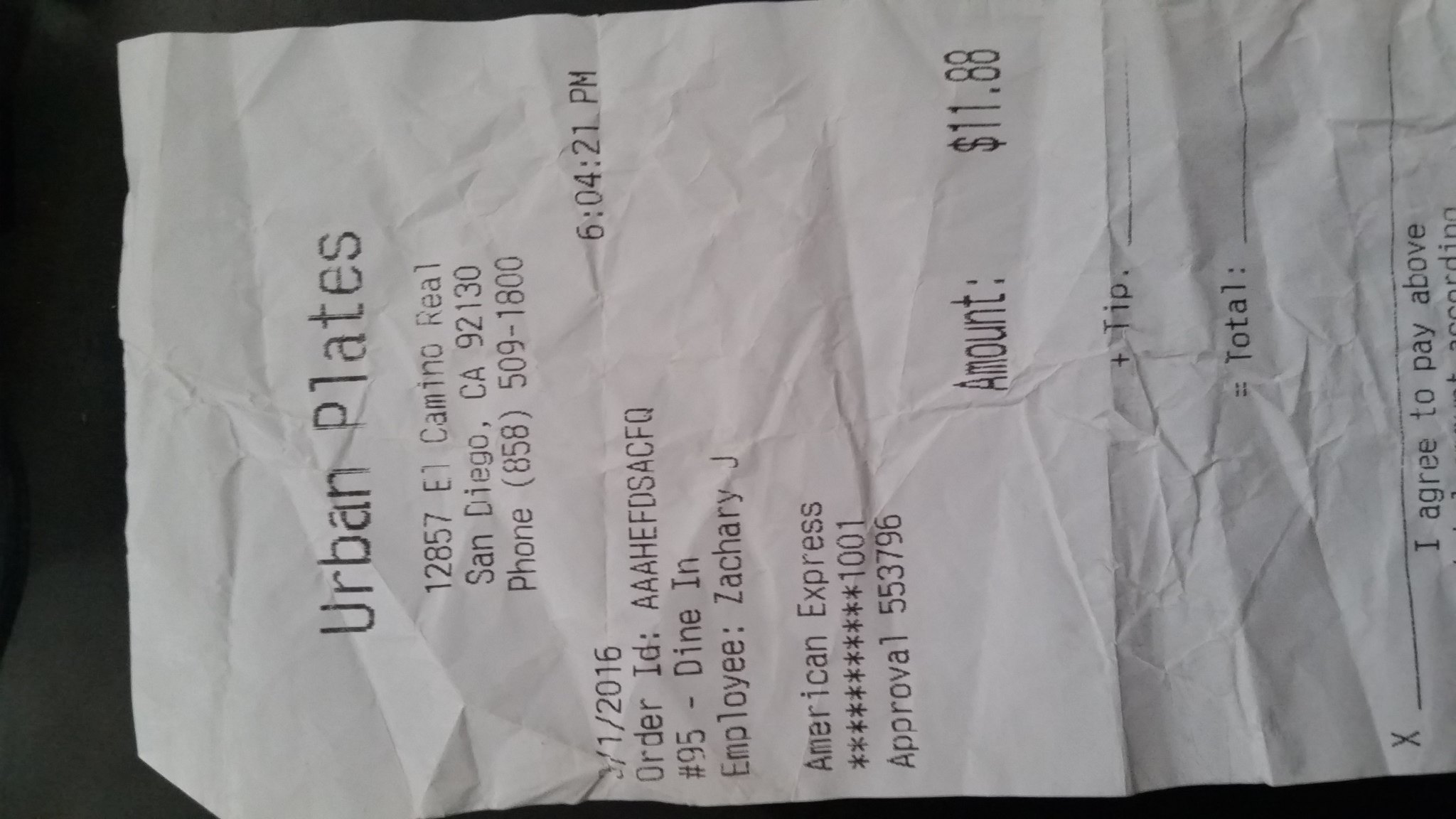This image shows a slightly angled receipt from Urban Plates, a dine-in restaurant located at 12857 El Camino Real, San Diego, California, 92130. The contact number listed is 858-509-1800. The receipt, dated March 1, 2016, at 6:04:21 p.m., was issued for an $11.88 transaction paid with an American Express card. The receipt indicates the employee's name as Zachary J. It is noted that the sections for the tip and total were left blank, suggesting this might be a customer copy. The order is identified as dine-in number 95, and an alphanumeric order ID "AAHEFDsACFQ" is printed.